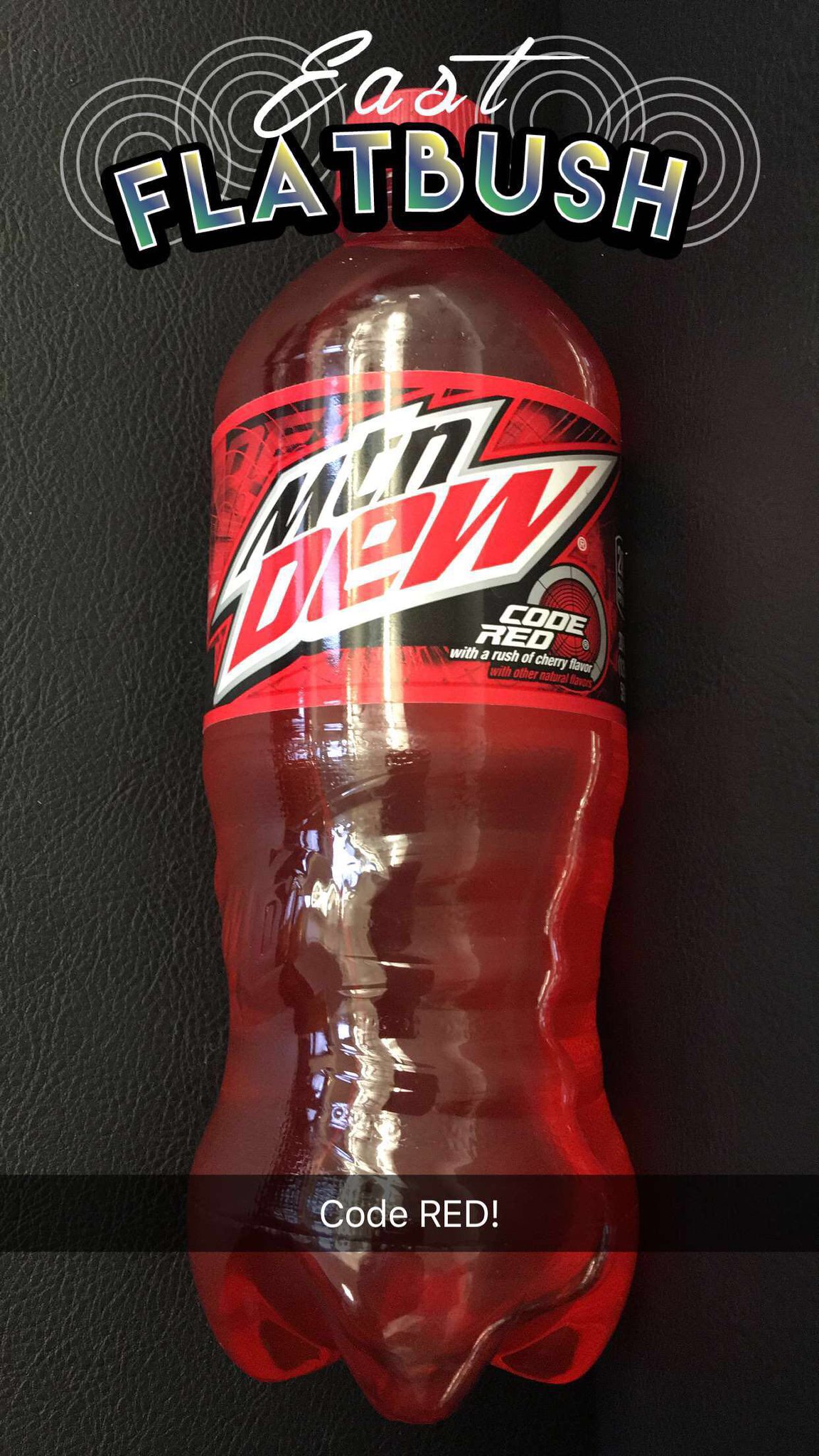The image features a stark black background with the word “EAST” prominently displayed in crisp white text. Beneath this, the word “FLATBUSH” appears in bold white letters, each letter outlined in a striking blue. The entire scene is dotted with numerous small white circles, creating a textured backdrop.

Front and center in the image stands a bottle of Mountain Dew Code Red. The bottle is adorned with a vivid red label. The brand name "MOUNTAIN" is printed in bold black letters at the top of the label, while "DEW" is immediately underneath in eye-catching red letters. Just below that, the specific product name "Code Zero" is clearly visible in white text. At the very bottom of the label, there's a black stripe running horizontally, containing the words "CODE RED" in white lettering. The bottle contains the distinctively red-colored Mountain Dew, indicating it’s a flavored variant of the popular beverage.